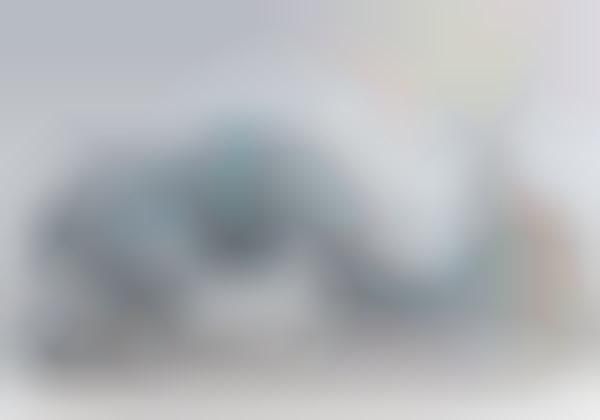The image presents an abstract, highly out-of-focus composition that conveys the feeling of a morning haze when vision is unclear and indistinct. The background consists of varying shades of white and gray, contributing to the overall blurry atmosphere. Prominently, there is a central blurb shaped like an 'S' curve, which starts as a gray color and transitions into a greenish hue, accentuated by a dark black oval shape at its lower part. This central blurb further morphs into a blue shade that lightens towards the right, continuing into another curvy line resembling a 'J'. This 'J' shape transitions through black, green, and light blue hues. Additionally, at the upper right, there is a faint yellow circular haze, while towards the bottom left, near the center, there is a circular shape outlined in black with teal accents. The image, devoid of any text, leaves a lot to the imagination, as the abstract forms and blurred colors blend together, making any object difficult to discern clearly.